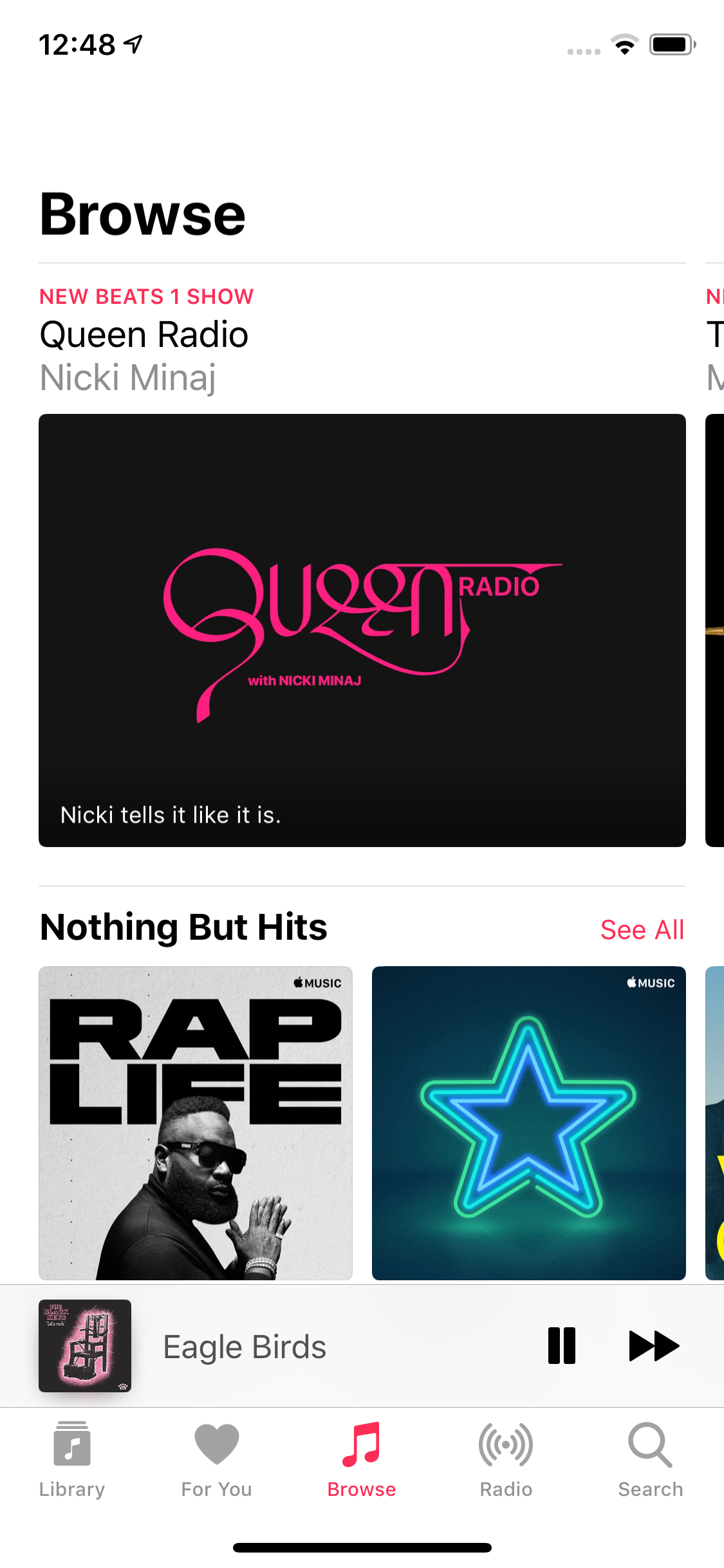The image depicts a cell phone screen with a user interface of a music streaming app. 

- The top left corner displays the time as 12:48, while the top right corner shows a fully charged battery icon.
- Below the status bar, the screen reads "Browse" in standard text.
- Prominently displayed in pink text is the phrase "New Seats or New Beats & One Show."
- Below this, "Queen Radio" is written in black text, followed by "Nicki Minaj" in gray text.
- The cover art directly underneath is predominantly black with "Queen" written in pink text at the center.
- Just below the cover art, there is a text that reads "Nothing But Hits" in black text, with a "See All" button to the right.
- Below, two album covers are featured side by side:
  - The left album cover is titled "Rap Life" and shows an artist from a side view with hands together in a prayer-like gesture.
  - The album cover on the right features a blue star in the center and is labeled with the song "Eagle Birds," which is currently playing.
- Further down, five icons are visible for navigating the app:
  - From left to right: Library, For You, Browse (highlighted in red), Radio, and Search.
- At the very bottom of the screen, there's a small horizontal black bar centered at the bottom.
- The overall background color of the screen is white.